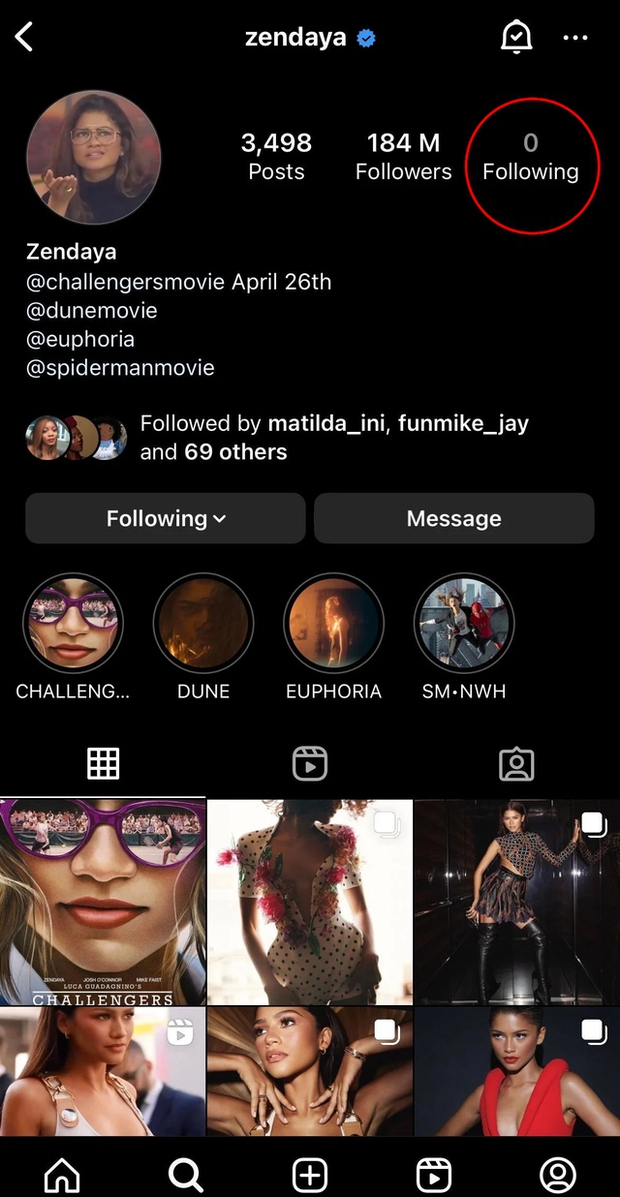Screenshot of Zendaya's Verified Instagram Page

This is a detailed screenshot of celebrity Zendaya's verified Instagram profile. At the top of the page, her name, "Zendaya," is prominently displayed with a blue checkmark beside it, indicating the account's authenticity. Zendaya's profile picture, shown within a circular frame, features her wearing glasses, holding her hand out seemingly to underscore an important point. 

The profile statistics reveal that Zendaya has made an impressive 3,498 posts. She boasts an astounding follower count of 184 million, while notably following no one, with the zero highlighted by a red circle.

Beneath her profile picture and name, there is a list of some of the major projects she has been involved in, accompanied by the "@" symbol:

- @ChallengersMovie (Release Date: April 26)
- @DuneMovie 
- @Euphoria
- @SpiderManMovie

Additionally, the screenshot includes a "Followed by" section, showcasing mutual connections — users who follow both Zendaya and the viewer. These include "Matilda_I_and_I," "FunMike_J," and 69 others.